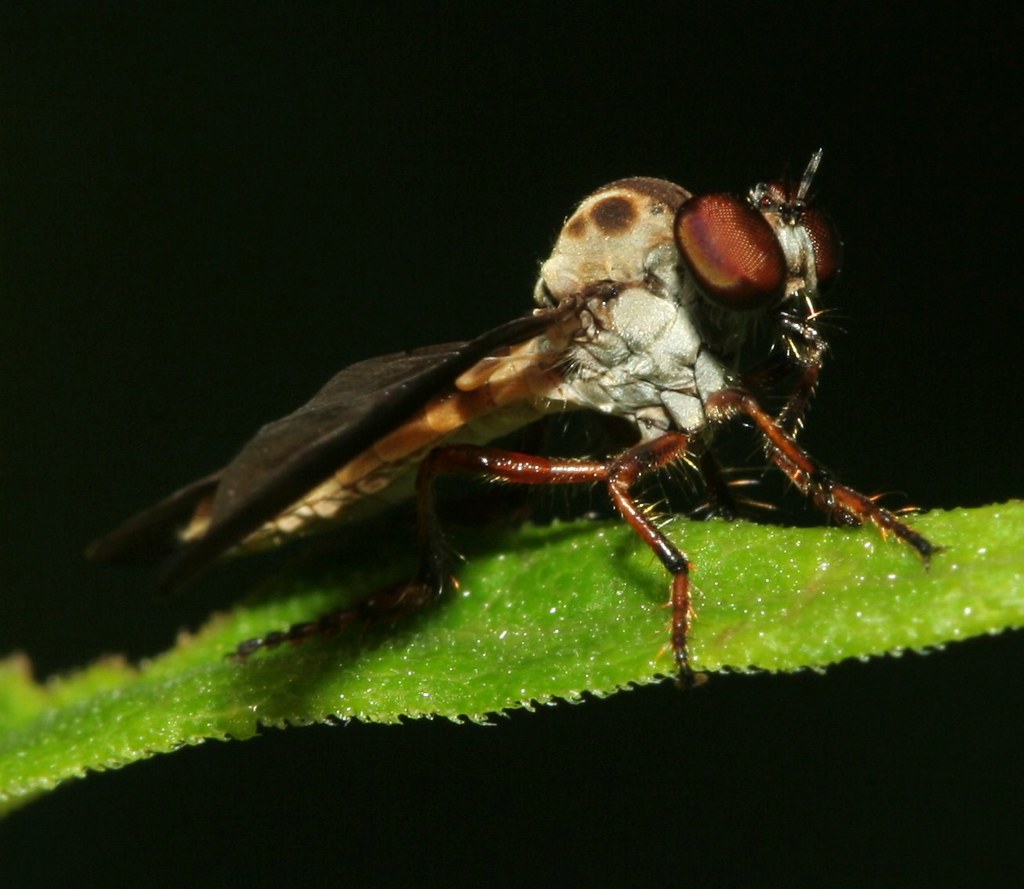The image captures a detailed close-up of an insect perched on a green leaf. The leaf, characterized by its bright, forest-green color and multiple fingerings, sharply contrasts with the dark, black background, suggesting the photograph might have been taken at night. The insect, facing to the right, exhibits a rather grotesque appearance, with distinct and varied shades of brown spread across its body. Its head features large, elliptical orange eyes and noticeable black mandibles, with what seems to be a small horn or antler-like structure. The creature's legs are long, hairy, and brown with black markings. Its body, segmented into a pronounced thorax and a white-bellied abdomen, extends into a long, thin tail. The insect's black and brown wings are extended, giving the impression of a moth at rest, though its species remains uncertain. Overall, the image emphasizes the striking details of this sizable and atypical moth-like insect against the stark simplicity of the leaf and the dark backdrop.